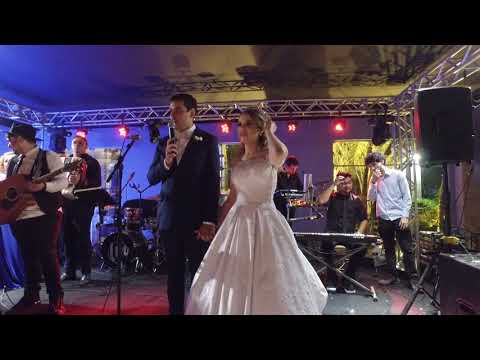In this detailed photograph, a bride and groom are the focal point, suggesting it's a wedding scenario. The groom stands to the left, clad in a dark blue suit with a white shirt and a neatly folded kerchief in his pocket. His dark hair is neatly trimmed as he holds a microphone close to his mouth, likely delivering a thank-you speech. The bride, slightly shorter, stands to his right in a beautiful white wedding dress. She has blonde hair and is holding the groom's hand with her right hand while adjusting her hair with her left. 

Behind the couple, a band is assembled, enhancing the celebratory atmosphere. Closest to the couple on our left is a guitarist wearing a top hat, suggesting a somewhat whimsical style. Further back and to the right, at least one keyboardist can be seen along with other instrumentalists, possibly another guitarist and a drummer, contributing to the musical backdrop. The lighting setup includes track lighting and mounted speakers, some casting a red hue, indicating a well-organized space for both the performance and the event. Additional people, possibly other musicians or attendees, are visible, adding to the lively ambiance of the small room.